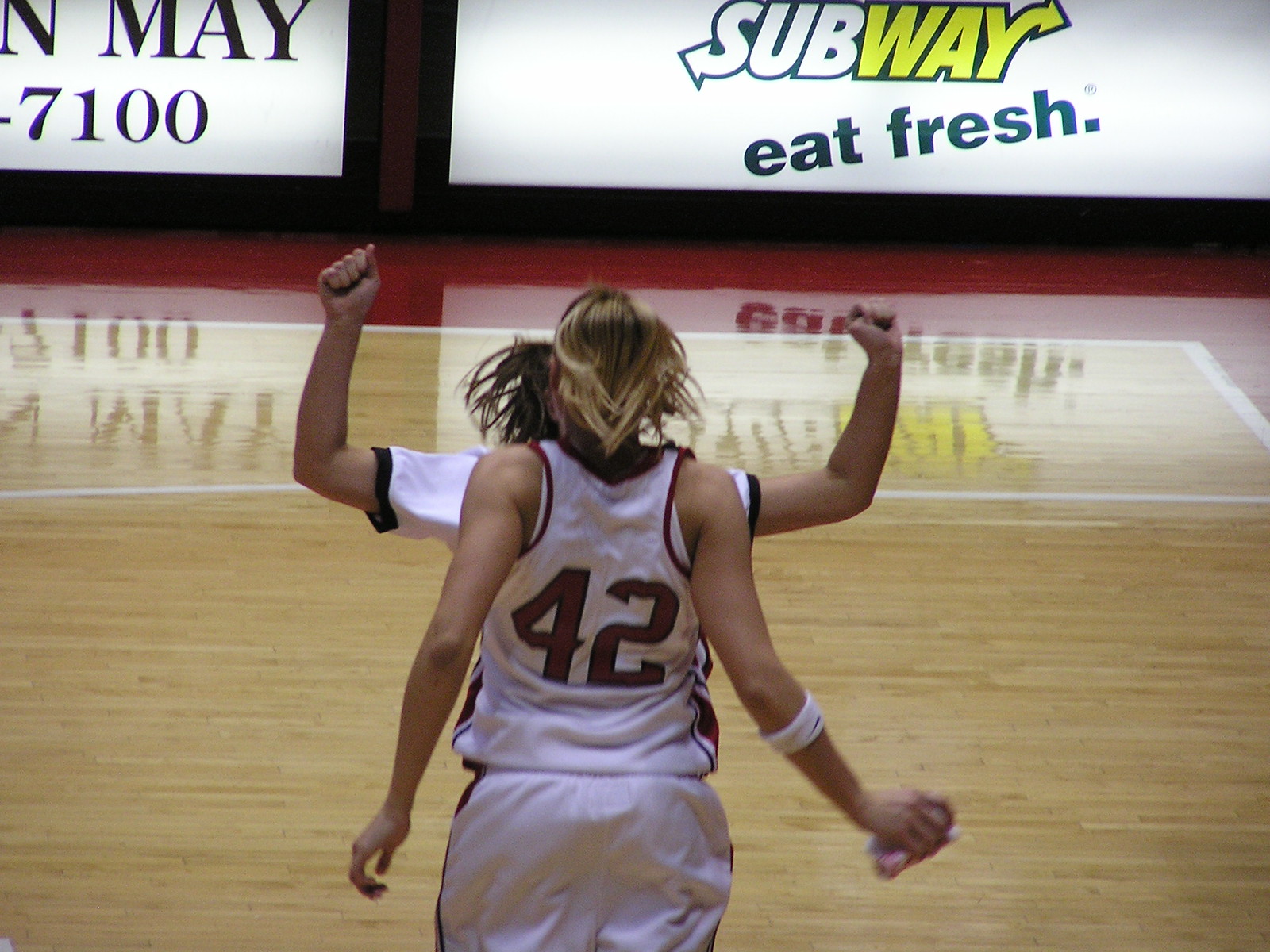In this detailed photograph, two women athletes are engaged in a chest bump on an indoor basketball court. The court has a polished light brown wooden floor marked with white lines and is bordered by a red out-of-bounds area. In the foreground, the first player is seen from the back. She has blonde hair pulled back into a ponytail and is wearing a white basketball uniform with red trim, sporting the red number 42 on her back. She also wears a white wristband on her right forearm and is holding an object in her right hand. Directly in front of her is another player, presumably African-American, whose face is obscured but whose darker skin and raised arms are visible. Both of her hands are clenched into fists, suggesting a defensive stance. This second player is dressed in a white short-sleeve shirt with blue trim. 

In the background, several advertising banners can be seen. To the right, on a white backdrop, is a Subway advertisement featuring the iconic green and yellow logo with the slogan "Eat Fresh" underneath. Another partially visible banner in the upper left corner displays black text with the partially readable words "May 7100." Both banners are securely framed with heavy black borders. The red zone bordering the wooden court appears designated for player and coach movements without interfering with on-court play.